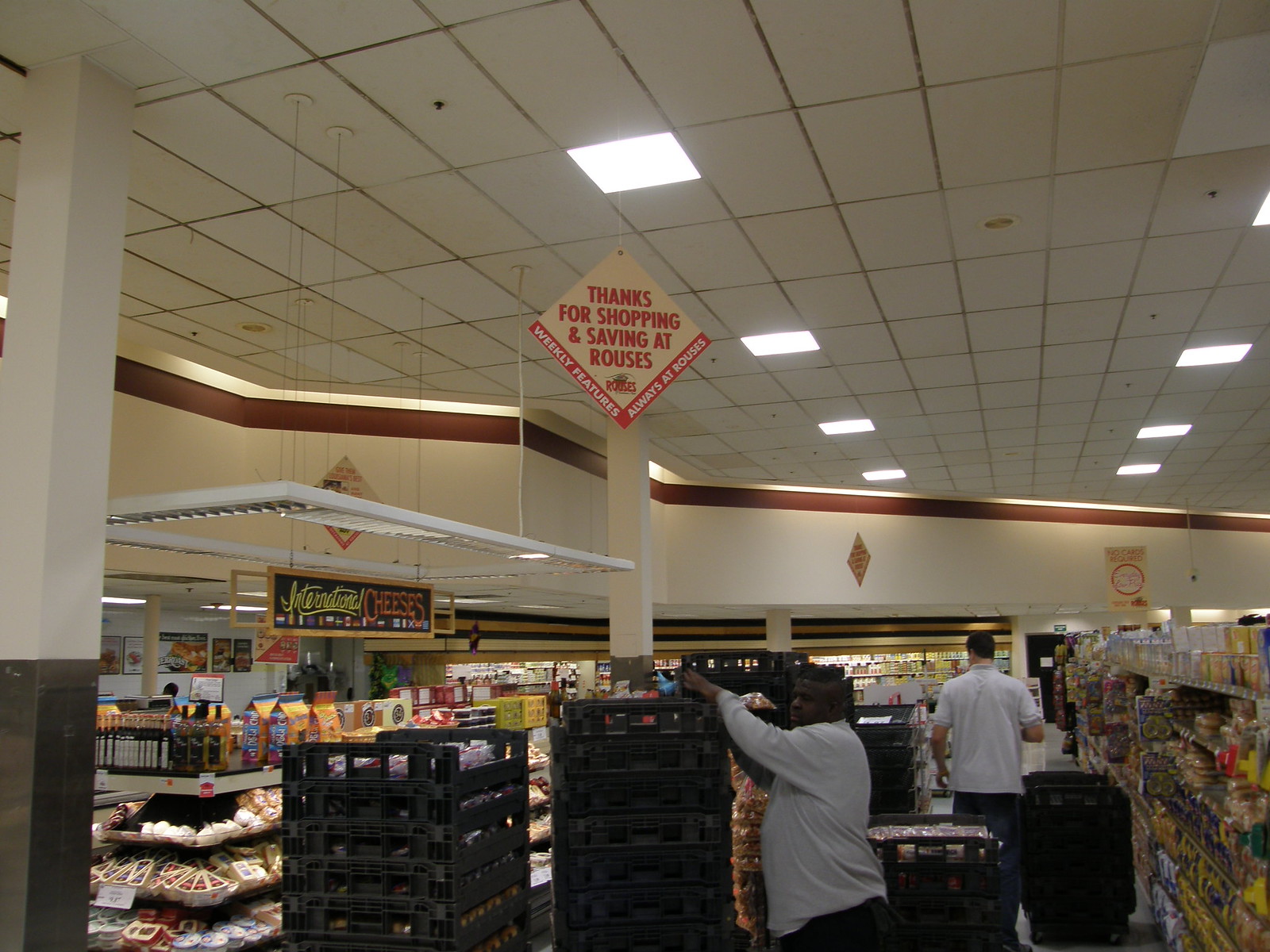This detailed image depicts the interior of a grocery store, where several individuals are visible amid the store's well-lit ambiance. The ceiling is designed with white, square-like panels featuring bright, square-shaped lights. Centrally hanging from the ceiling is a diamond-shaped sign that reads, "Thanks for shopping and saving at Rouses," with additional text indicating "Weekly features" on the left and "Always at Roses" on the right. In the foreground, a man, clearly a black individual with very short hair and slightly heavy, is taking items out of tall, stackable gray plastic trays. Nearby, a Caucasian man, presumed to be shopping, is walking away alongside some racks filled with bread and possibly boxed items. The shelving units feature angled, recessed shelves showcasing various cheeses, highlighted by a handwritten wooden sign that reads "International Cheeses." In the background, a bank of refrigerators, likely containing beverages and other perishable items, lines the wall. The organized layout and activity convey a bustling atmosphere typical of a supermarket.